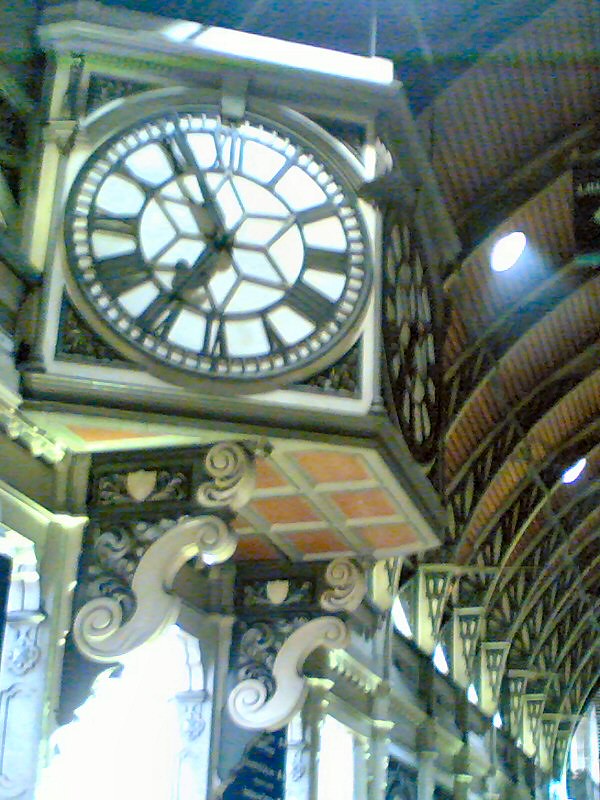This color photograph, slightly out of focus and grainy, depicts an interior scene reminiscent of a historic train station. Dominating the upper portion of the image is a large, curved ceiling featuring high arches and small, round skylights. The room is bathed in natural light flooding in from windows at the bottom of the frame. The most prominent feature is an ornate, old-fashioned wall clock with Roman numerals, which displays the time as five minutes to seven. This black and white clock, adorned with a six-pointed star at its center, is set against a backdrop of intricate, old-timey architectural details. The photograph, taken at a low angle looking up, emphasizes the grandeur and vintage charm of the space while leaving the lower portions and ground level of the building out of view. There are no people, animals, plants, or additional writings visible in the image, and its vertical composition accentuates the towering elegance of the scene.